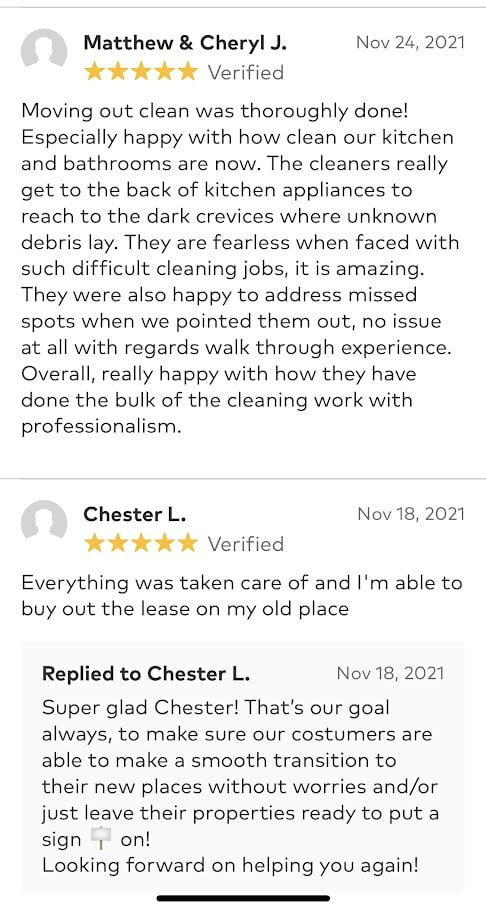**Customer Testimonials: Exceptional Move-Out Cleaning Service**

**Matthew and Cheryl J. - Verified 5-Star Review (November 24th, 2021)**
"Our move-out cleaning was thoroughly done, and we were especially happy with how clean our kitchen and bathrooms are now. The cleaners went above and beyond, reaching the back of kitchen appliances and tackling the dark crevices where hidden debris often accumulates. Their fearless approach to difficult cleaning jobs was truly impressive. Additionally, they were more than willing to address any missed spots we pointed out, ensuring our complete satisfaction. The walk-through experience was seamless, and overall, we are extremely pleased with the professional and meticulous work they put into making our home spotless."

**Chester L. (November 2021)**
"Everything was taken care of, and I am now able to buy out the lease on my old place. The service ensured a smooth transition with no worries."

**Response to Chester L.**
"Super glad, Chester. That's our goal: to ensure our customers can smoothly transition to their new places without worries or leave their properties ready to sell. Looking forward to helping you again."

---

These testimonials highlight the dedication and professionalism our cleaning team brings to their work, ensuring every customer has a worry-free experience during their move-out process.